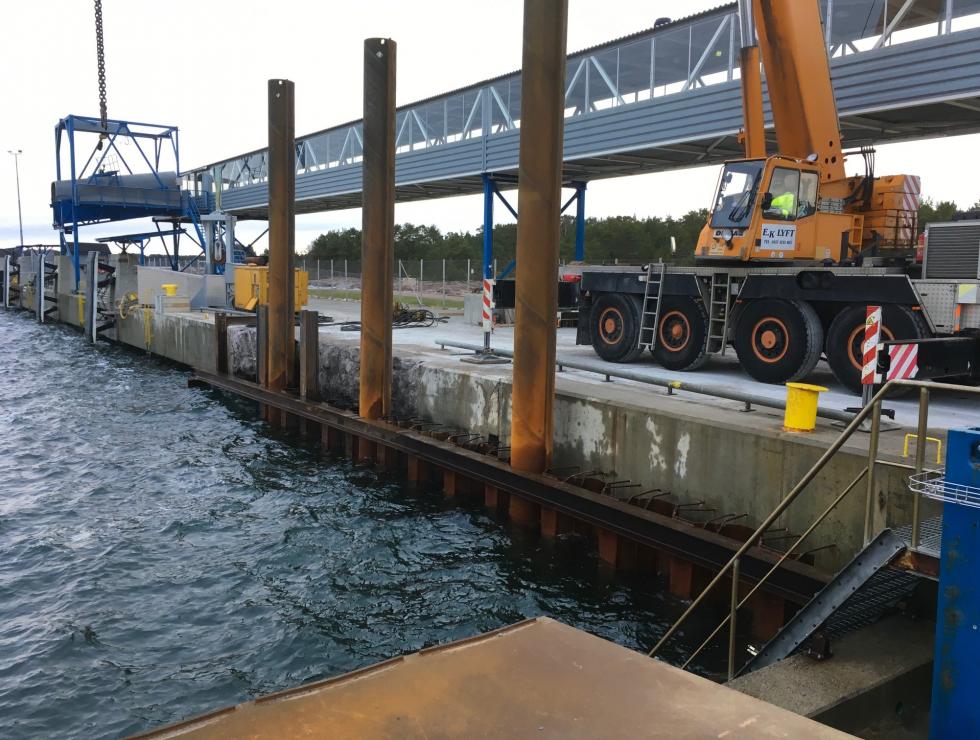The image depicts an active construction site situated on the edge of a dock. In the bottom left of the frame, there is a body of water adjacent to a large concrete slab where construction work is ongoing. In the middle of this slab, a driving path for construction vehicles is visible, featuring a large truck equipped with a crane. A giant heavy industrial chain lifts items in the background. To the top right, a covered walkway structure spans across the frame. Three rusty, brown support struts are also visible, adding to the industrial atmosphere. The color palette of the image includes shades of white, blue, yellow, brown, red, and lime green, and there is no text visible except on the construction vehicles. The scene captures the bustling activity of the construction process against the backdrop of the sky.